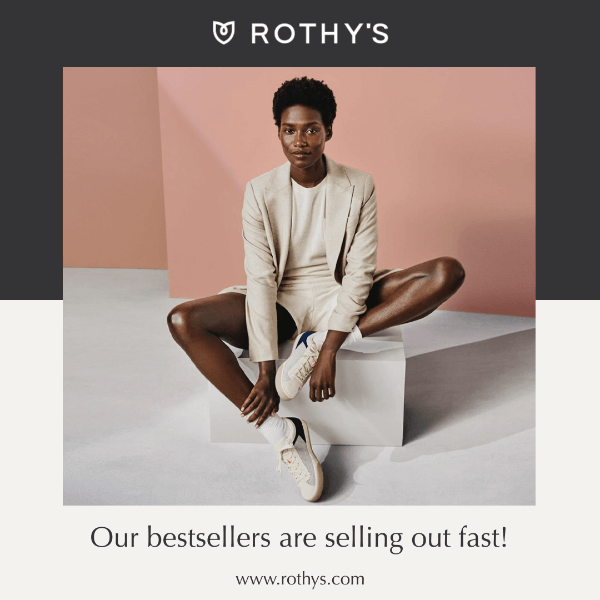This is a screenshot of an advertisement for a business called Rothy's, stylized as "R-O-T-H-Y Posh V-S." To the left of the name, there is an icon resembling a shield with a circle in the center. Both the Rothy's text and the shield icon are rendered in white ink. The top half of the ad features a black background, while the bottom half is white.

In the center of the ad, there is an inset picture. The upper section of this inset showcases a pink wall, while the lower section displays a light gray or white floor. A slender black woman with short, curly black hair sits on a white block within this inset. Her facial expression appears indifferent. She is dressed in a long-sleeved, beige business jacket and a matching thin-material outfit that looks like a one-piece shorts set. Her legs are bare, and she wears white socks and white tennis shoes that have a black detail at the back.

Below the inset, there is a caption that reads, "Our best sellers are selling out fast!" Followed by the website URL, "www.rothys.com."